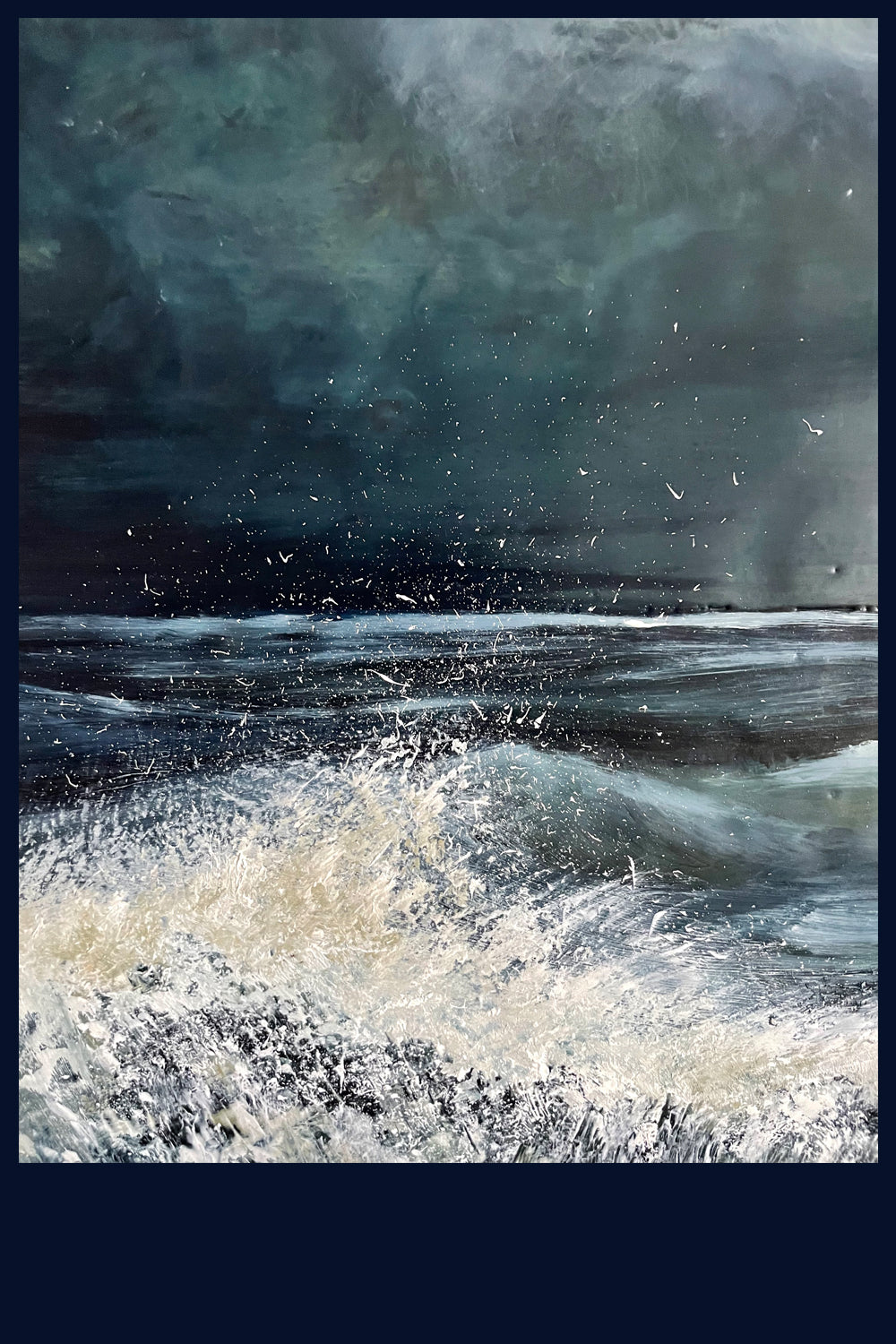The painting portrays a tumultuous nature scene with an almost surreal, painterly quality, evidenced by visible brush strokes in the ominous sky. The foreground is dominated by the drama of whitewater rapids, the river appearing swollen from rainfall, with water crashing and splashing vigorously. Waves are distinct, both near and afar, creating a sense of continuous motion and power. The sky above is laden with dark, stormy clouds tinged with hints of purple, blue, and green, contributing to the menacing atmosphere. The scene is enveloped in darkness, with hues varying from almost pitch black on the left to slightly lighter shades towards the top. A noticeable feature is a black banner-like area around the waves, enhancing the contrast and drama of the whitewater against the dark, stormy seas and sky. Scattered throughout are splashes of water resembling large shards, adding to the chaotic energy of the scene. This painting captures a raw, powerful moment in nature, where the elements clash dramatically.